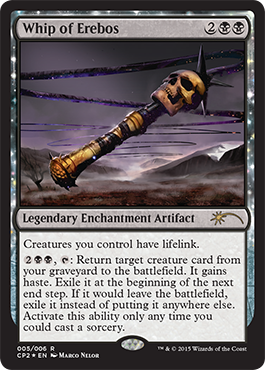This image features a card from the card game Magic: The Gathering. The card, appearing to be a common type received from standard card packages, is set against a predominantly black background with a shimmering silver border. 

At the top of the card, the item is identified as "Whip of Erebos" written in black text. Adjacent to this is the card’s mana cost, indicated by a “2” followed by two icons resembling stars within circles.

The centerpiece of the card is an illustration of the Whip of Erebos. The whip is depicted as having a handle that is gold and black, topped by a yellowed human skull. A black whip extends from the skull, disappearing into the background. The background itself is dark and foreboding, featuring a deep purple sky with ominous clouds, rugged mountains, and barren terrain. A dead tree is distinctively visible on the left side of the scenery, enhancing the desolate atmosphere.

Beneath the illustration, the card identifies the object as a "Legendary Enchantment Artifact." Further down, within a white rectangle with black text, the card details the artifacts’ abilities: "Creatures you control have lifelink. Return target creature card from your graveyard to the battlefield. It gains haste. Exile it at the beginning of the next end step. If it would leave the battlefield, exile it instead of putting it anywhere else. Activate this ability only any time you could cast a sorcery."

At the very bottom of the card, additional information is provided in white text against a black background, further clarifying the card's features and rules.